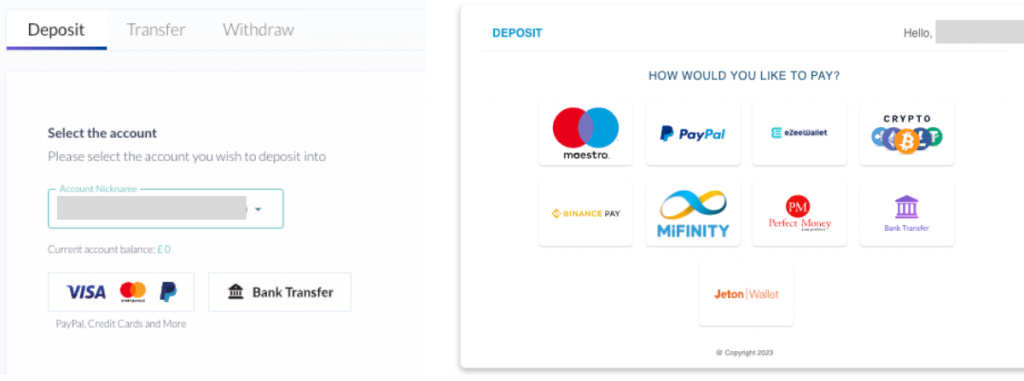The image displays an online banking interface with several interactive elements. At the top left corner, the word "Deposit" is prominently highlighted in blue, indicating the active action. To the top right, there's a gray box labeled "Hello," but it does not display a name.

Central to the image are two vertical sections. The left section first presents three options: Deposit, Transfer, and Withdraw. Under the highlighted "Deposit" option, a prompt says "Select the account" with a drop-down box for account nicknames beneath it. It also displays the current account balance, which is zero euros.

Below the account balance are two options for payment methods on the left: Visa, MasterCard, PayPal, and Bank Transfer. Adjacent to this, the right section holds a large box centrally labeled "How would you like to pay?" within which are two rows of payment icons. The first row includes Maestro, a blue and red overlapping circle, the PayPal logo, Easy Wallet, and a Crypto option. The second row contains Binance, Binance Pay, Mifinity, Perfect Money, and a bank transfer icon. Centered below these is a single option labeled Jeton Wallet.

The entire interface has a clean, white background with white boxes for each option, ensuring a user-friendly and straightforward design. At the bottom of the image, a "Copyright" notice is visible.

Overall, the interface provides a simple, intuitive layout for users to make a deposit, showcasing various payment methods and clear navigation options.